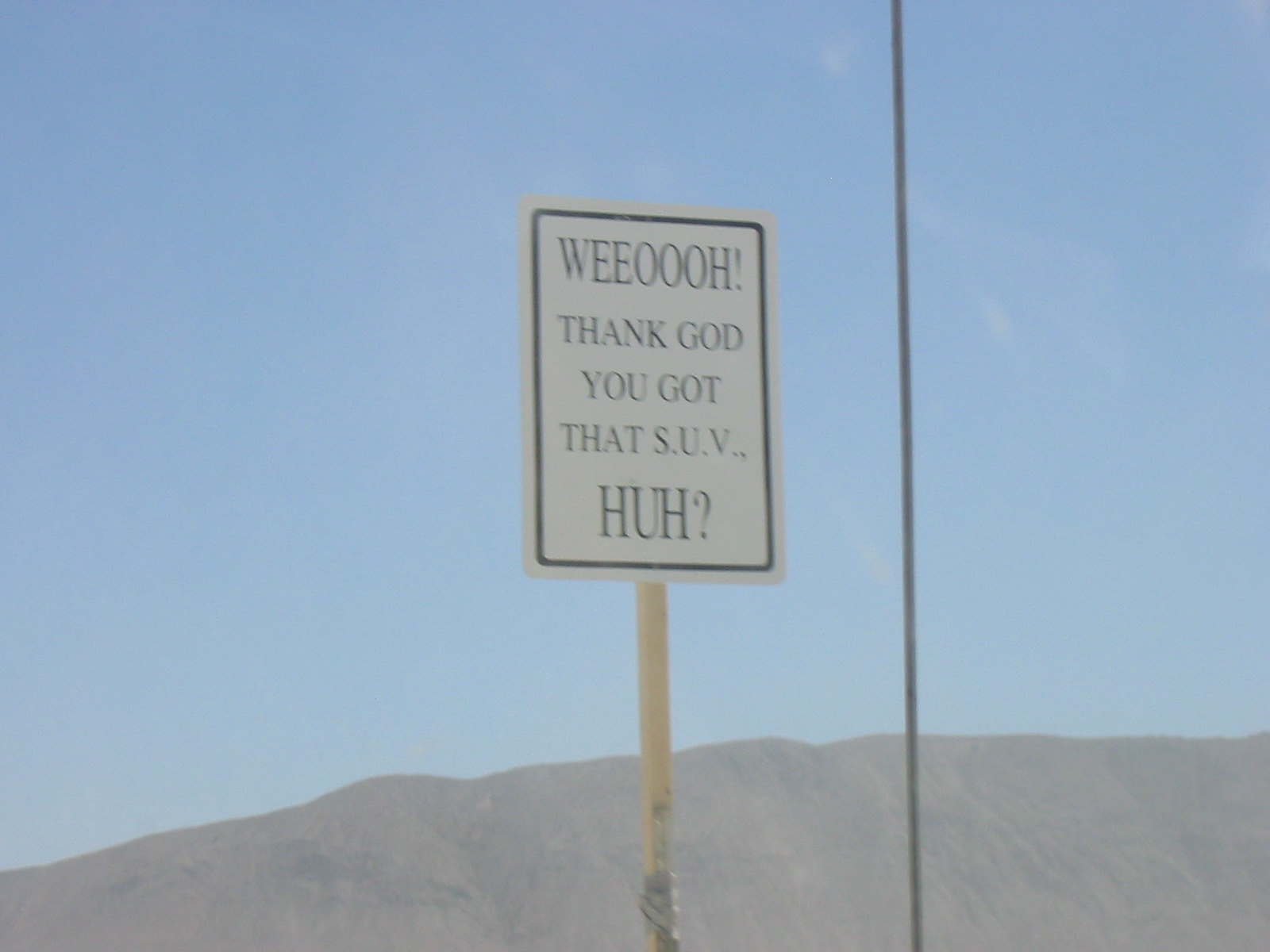The photograph captures a roadside scene dominated by a white sign featuring black text on a yellow steel pole with some rust at the bottom. The sign humorously reads, "Weeoooh! Thank God you got that SUV, huh?" Adjacent to the sign is a long black wire that extends from the top to the bottom of the image. The background reveals a striking, clear blue sky with a faintly gray cast over the entire image, suggesting it might have been taken through a window. Below the sky, a mountainous landscape stretches across the bottom of the frame, showcasing brown and black hues. The scene is devoid of traffic or additional elements, emphasizing the humorous sign against the serene and slightly surreal outdoor setting.